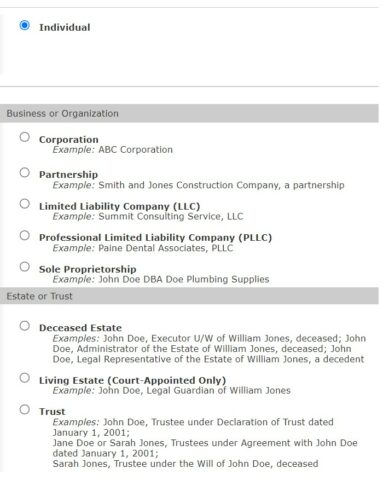This image illustrates a detailed hierarchical structure chart of various organizational and individual entity types. The diagram features three main grey divisions interconnected by lines. The top section, representing individual membership, features a blue-outlined circle labeled "Individual." 

Below this, a grey rectangle marks the beginning of the "Business or Organization" section. Within this section, there are several nested circles, each representing different types of business entities:

- A circle labeled "Corporation" with an example: "ABC Corporation".
- A circle labeled "Partnership", exemplified by "Smith and Jones Construction Company, a partnership".
- A circle for "Limited Liability Company (LLC)" with the example "Submit Consulting Services, LLC".
- A circle for "Professional Limited Liability Company (PLLC)" illustrated by "Paying Dental Associates, PLLC".
- Another circle titled "Sole Proprietorship", with the example "John Doe DBA Doe Plumbing Supplies".

Underneath this, a second grey rectangle indicates the "Estate or Trust" section. This section includes:

- A circle titled "Deceased Estate" with the detailed example: "John Doe, Executor U/W of William Jones, deceased; John Doe, Administrator of the Estate of William Jones, deceased; John Doe, Legal Representative of the Estate of William Jones, deceased".
- A circle for "Living Estate (Court Appointed Only)", with the example "John Doe, Legal Guardian of William Jones".
- Lastly, a circle labeled "Trust" with multiple examples: "John Doe, Trustee under Declaration of Trust dated January 1, 2001; Jane Doe or Sarah Jones, Trustees under Agreement with John Doe dated January 1, 2001; Sarah Jones, Trustee under the Will of John Doe, deceased".

This structured diagram comprehensively categorizes the entities in a visually organized manner, providing clear examples for each type.